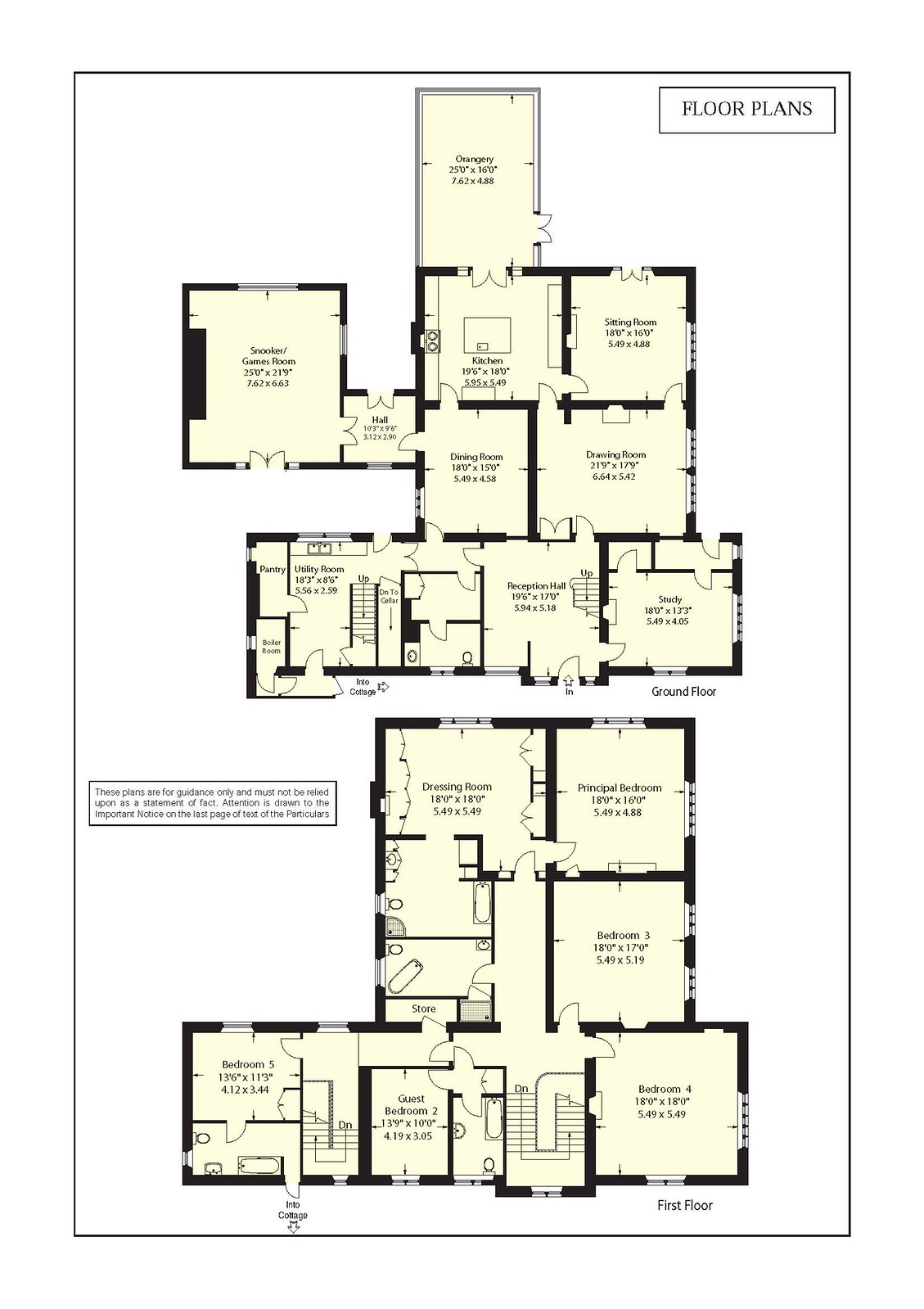This detailed floor plan illustrates a spacious, two-story European-style house. The ground floor layout is displayed at the top, while the first floor is depicted at the bottom. A disclaimer on the plan states: “These plans are for guidance only and must not be relied upon as a statement of fact. Attention is drawn to the important notice on the last page of text of the particulars.”

Entering from the ground floor, you are greeted by a gracious reception hall that grants access to a utility room and the staircase. Adjacent to the hall are a pantry and boiler room. On the right side of the plan, the layout features a study, drawing room, dining room, kitchen, sitting room, and an orangery. A hallway extends to a snooker/games room, providing a secluded area for recreation.

Ascending to the first floor, the design includes a dressing room and the principal bedroom, along with a couple of bathrooms. Five additional bedrooms are labeled: Bedroom Three, Bedroom Four, Bedroom Five, Guest Bedroom Two, and another guest bedroom. There are roughly three bathrooms dispersed throughout this level. The dual-sided staircase is prominently featured, while an additional set of stairs, positioned towards the left next to Bedroom Five, has its own bathroom. Both staircases appear to lead into an adjacent cottage, which is not depicted in the floor plans provided. This cottage serves as a distinct yet connected living area, extending the main house's functionality and space.